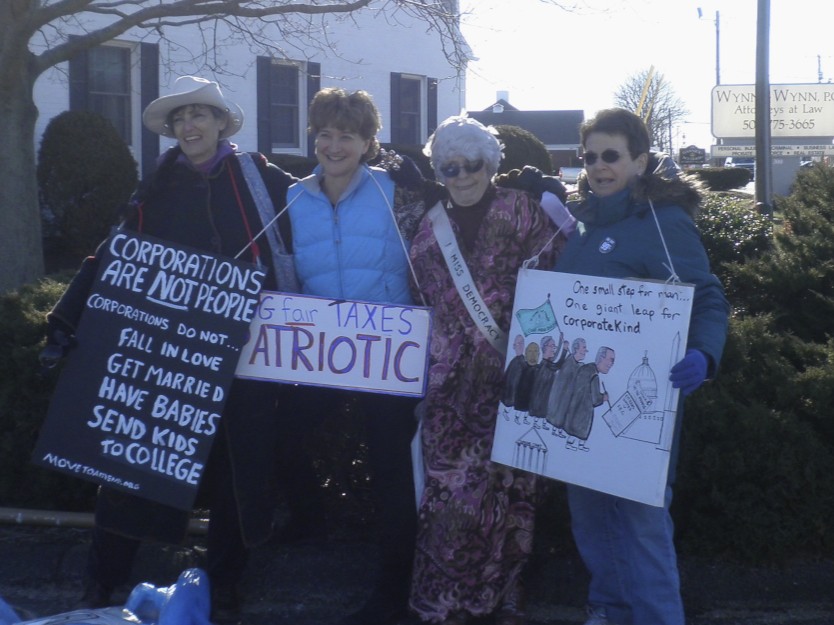In this outdoor, daytime photo taken in low lighting, four women of varying ages stand smiling in front of a white building with a sign that reads "Win-Win Attorneys at Law." Behind them are trees and bushes, including a leafless tree on the far left. The women, participating in a protest, wear signs draped around their necks with messages about corporations. One sign reads, "Corporations are not people. Corporations do not fall in love, get married, have babies, send kids to college." Another sign appears to be partly obscured, but you can make out "fair taxes" and "patriotic." The last sign states, "One small step for man, one giant leap for corporate kind," accompanied by a hand-drawn image of old men in black robes carrying a green flag near Washington D.C.'s monuments.